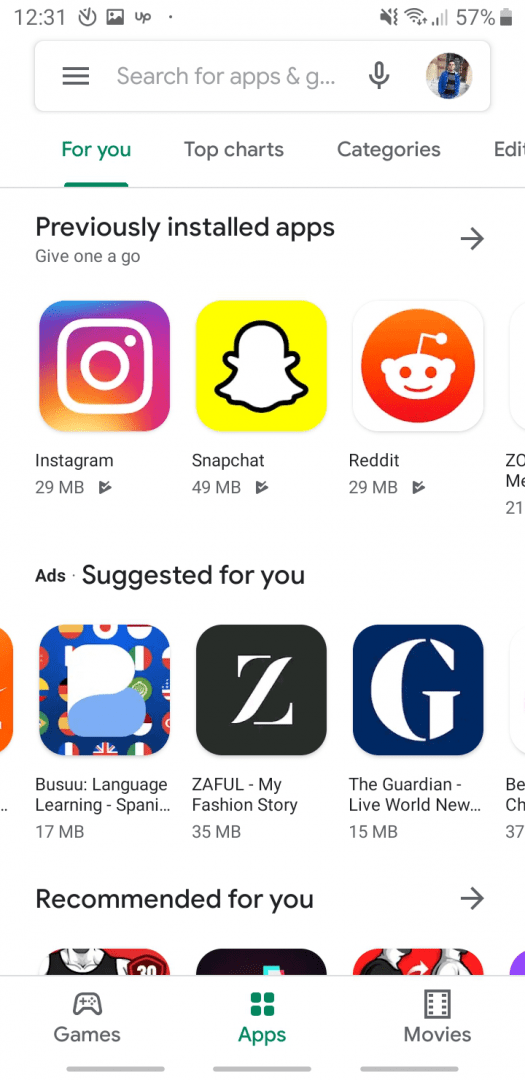A picture taken from a cell phone screen, displaying the time as 12:31 in the top left corner. In the top right corner, the battery icon indicates a 57% charge. Various icons are visible on both sides of the status bar. Below the status bar, the screen shows a search bar partially filled with the text "search for apps and G..." followed by a "For You" section. This section includes tabs for "Top charts," "Categories," "Edit," and "Previously installed apps," with the prompt "give one a go." Displayed apps include Instagram, Snapchat, Reddit, and an app partially cut off, possibly Zoom. Further down, an "Ads" section titled "Suggested for you" features Basu Language Learning (Spanish), Zaful (my fashion story), The Guardian (Live World News), and three more apps that are partially cut off at the bottom of the picture.